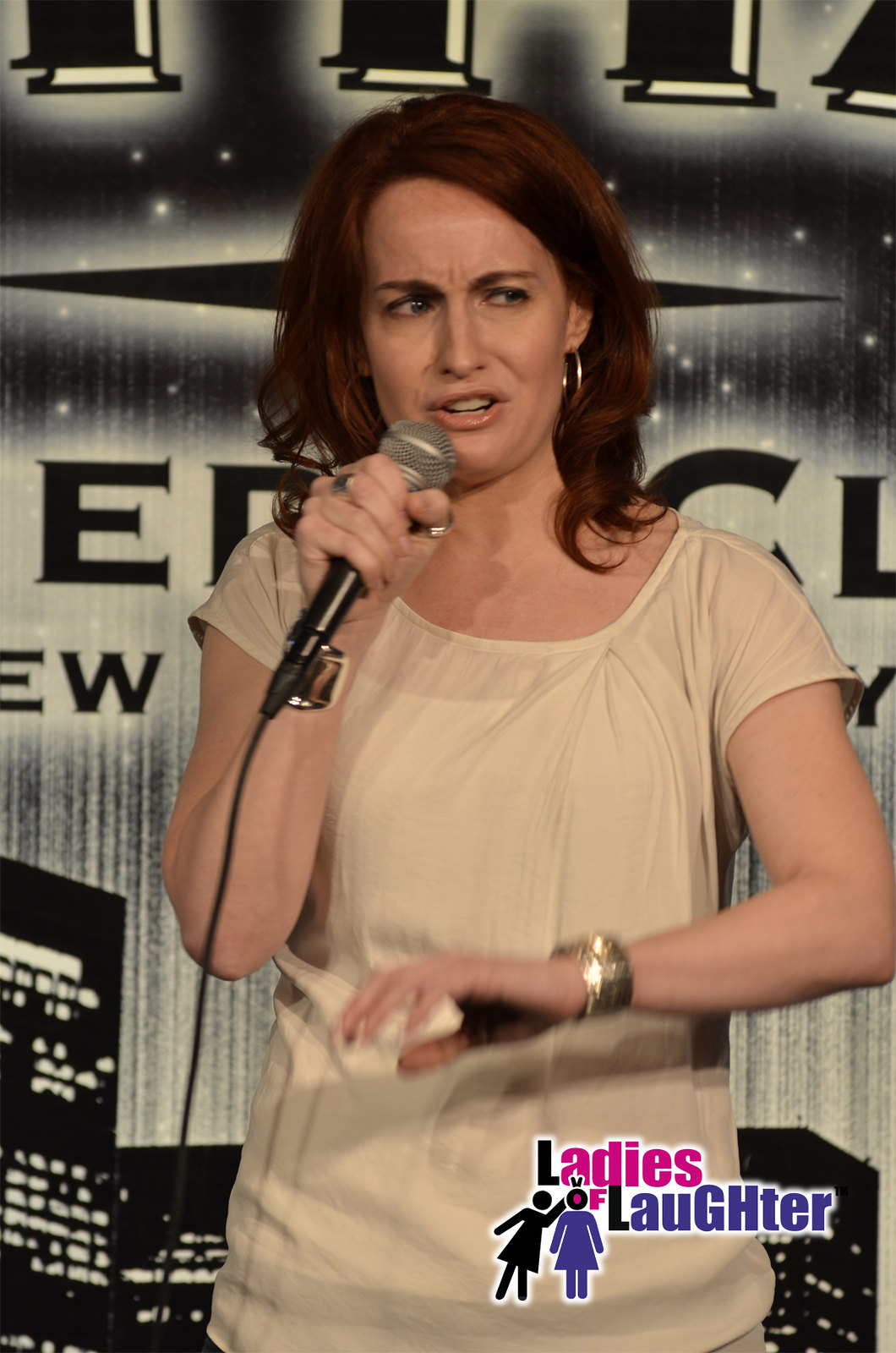This color photograph portrays a woman in her mid to late 30s standing on a stage, mid-speech, with a microphone in her right hand. She has medium-length, dark red hair and is wearing gold hoop earrings. Her face is animated and her mouth is open, indicating she is actively speaking. Her left hand is in motion, appearing blurred in the image. She is dressed in a short-sleeved beige shirt and accessorized with a gold or silver watch on her wrist and a ring on her left middle finger. The backdrop behind her resembles a nighttime cityscape with images of tall buildings, skyscrapers, and hotels illuminated against a starry sky. The setting evokes a comedy club or performance venue atmosphere. In the bottom right-hand corner of the photograph, the text "Ladies of Laughter" suggests that she is a female comedian performing at the time the photograph was taken.